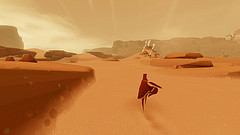The image, though small, captures a scene from what appears to be a gameplay session set in a desert landscape. A cloaked figure, draped in shades of burgundy with hints of gold, traverses the sandy terrain. The sand itself is a mix of tan and orangey-brown hues, with some small piles visible to one side. Particles of sand are seen blowing gently across the scene, adding to the sense of motion and desolation. Medium brown sand formations punctuate the foreground, giving texture to the barren expanse. The sky above is ominous, tinged with gray and marbled with faint cloud lines. In the distance, hills and rock formations break the horizon, adding depth to the panorama. The image quality is notably clear, with even the grainy texture of the sand distinctly visible.